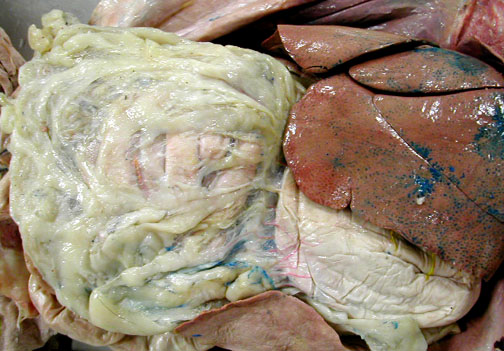This detailed color photograph is a close-up view of the internal organs of an animal, specifically showing a complex assortment of tissues and structures that are somewhat difficult to identify. On the right-hand side, there is a prominent organ that could be a liver, exhibiting a pinkish-bluish hue. Below and to the left of this organ appears to be the largest component in the image, possibly intestines or another large internal structure. The left side of the photograph displays what looks like a bluish-pinkish bag-like item that appears soft, potentially another organ or tissue. Scattered around the image, especially near the top right and bottom, are darker colored tissues, possibly skin, with hints of blue and red coloring, suggesting blood vessels or muscle tissue. Additionally, there is a white substance on the right side, enhancing the complexity and mysterious nature of the contents. The confusing and somewhat disturbing arrangement also includes elements resembling a seafood-like composition, potentially a hard-shelled crustacean such as a lobster or crab, with shiny, molded, and possibly plastic-wrapped bundles that look unnatural and alarming. This combination of various textures and colors contributes to the eerie and unsettling nature of the image, leaving one questioning if it is a genuine depiction of animal insides or an artificial, potentially hazardous construct.